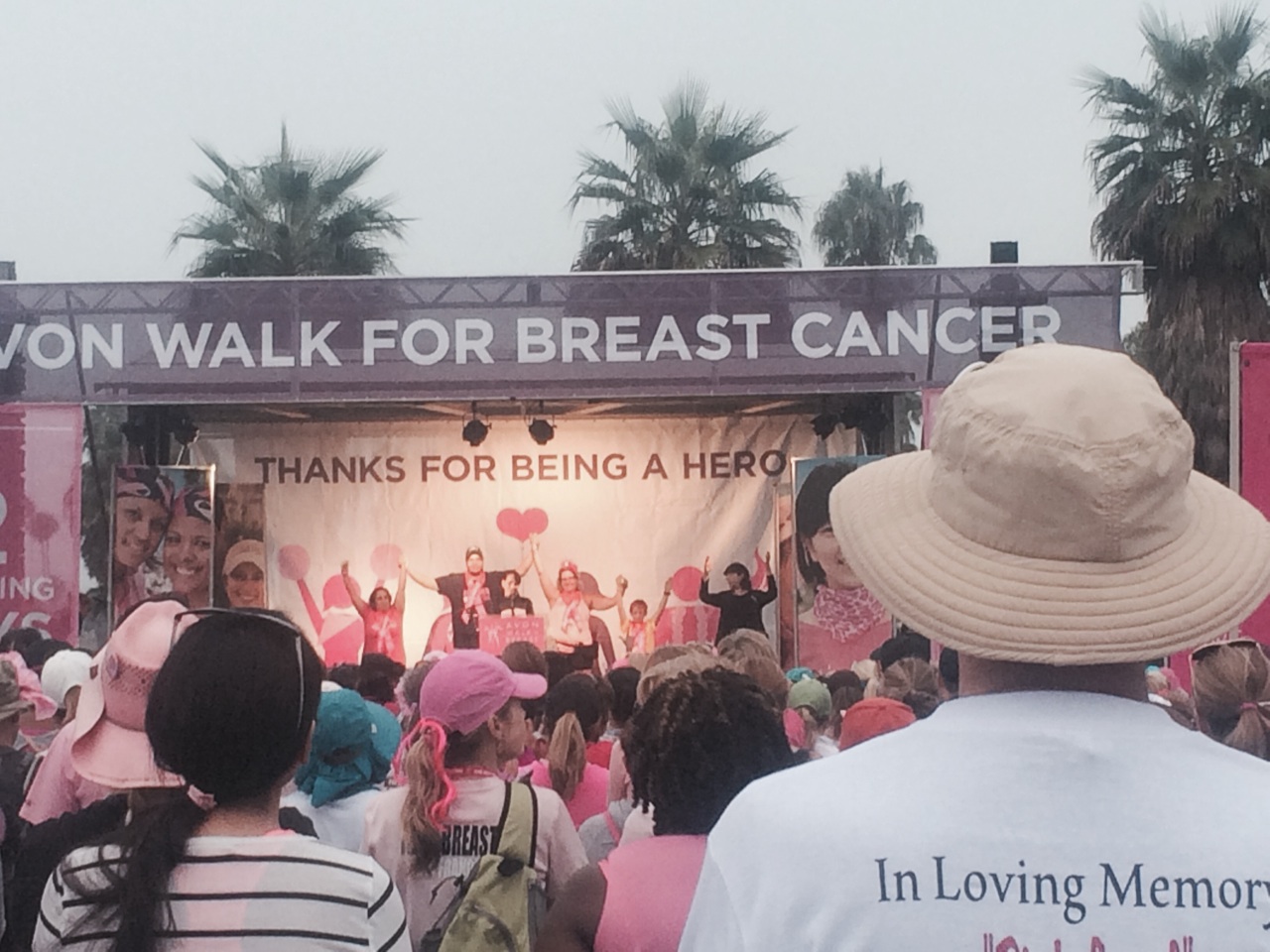The image captures a vibrant event centered around a breast cancer walk. A large stage is adorned with banners that proclaim "Walk for Breast Cancer” and “Thanks for Being a Hero," with a heart prominently displayed on the latter. On the stage, a diverse group of people—primarily women and including a small child—stand with their hands held together and raised triumphantly towards the sky. Surrounding the stage are several spectators. In the foreground, a man wearing a tan bucket hat and a white t-shirt with partial visible text "In Loving Memory" is noticeable. To his left is a woman with black hair pulled into a ponytail, dressed in a white shirt with black horizontal stripes, and glasses perched on her head. The scene is set outdoors, with palm trees visible against a slightly overcast sky, adding to the atmosphere of communal support and celebration. Many participants are clad in pink to show solidarity for the breast cancer cause.